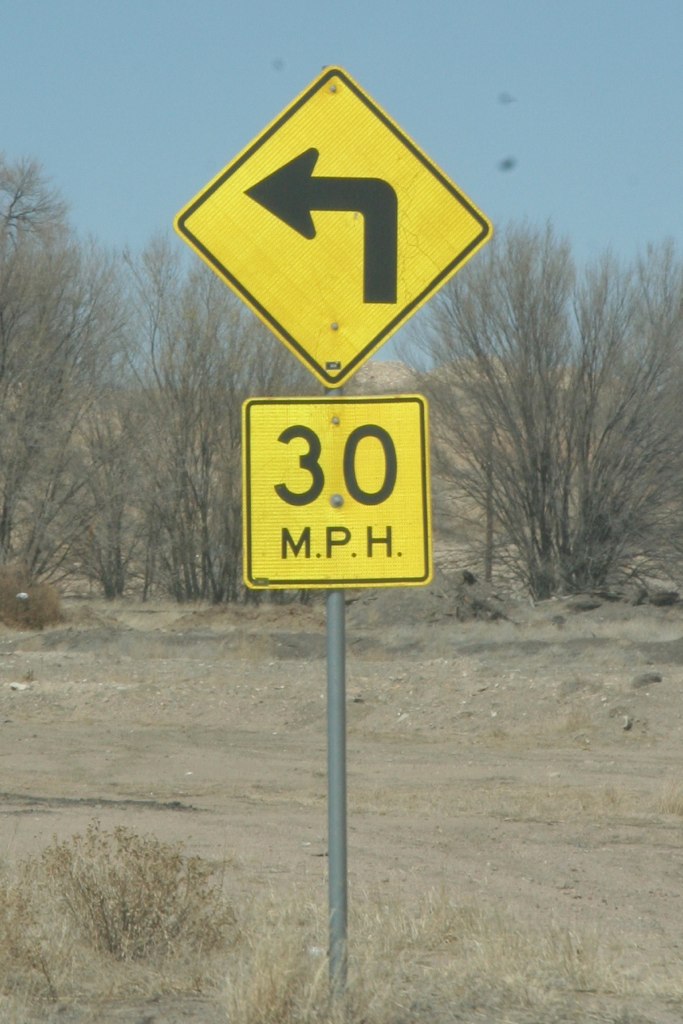The image features a street sign situated in what appears to be a semi-deserted area, bordered by sparse vegetation and tall, scrubby trees without leaves. The setting suggests a remote or coastal environment, potentially near a beach. The street sign consists of a silver pole. At its lower section, there is a rectangular sign indicating a speed limit of 30 miles per hour. Above it, fastened securely to the pole, is a yellow diamond-shaped sign with a black border, displaying an arrow that bends to the left, likely warning of an upcoming curve in the road. The sky above is clear, with a scattering of birds in flight, although some tiny specks might also be dust particles on the camera lens. The bright daylight enhances the starkness of the terrain and the prominence of the signage.